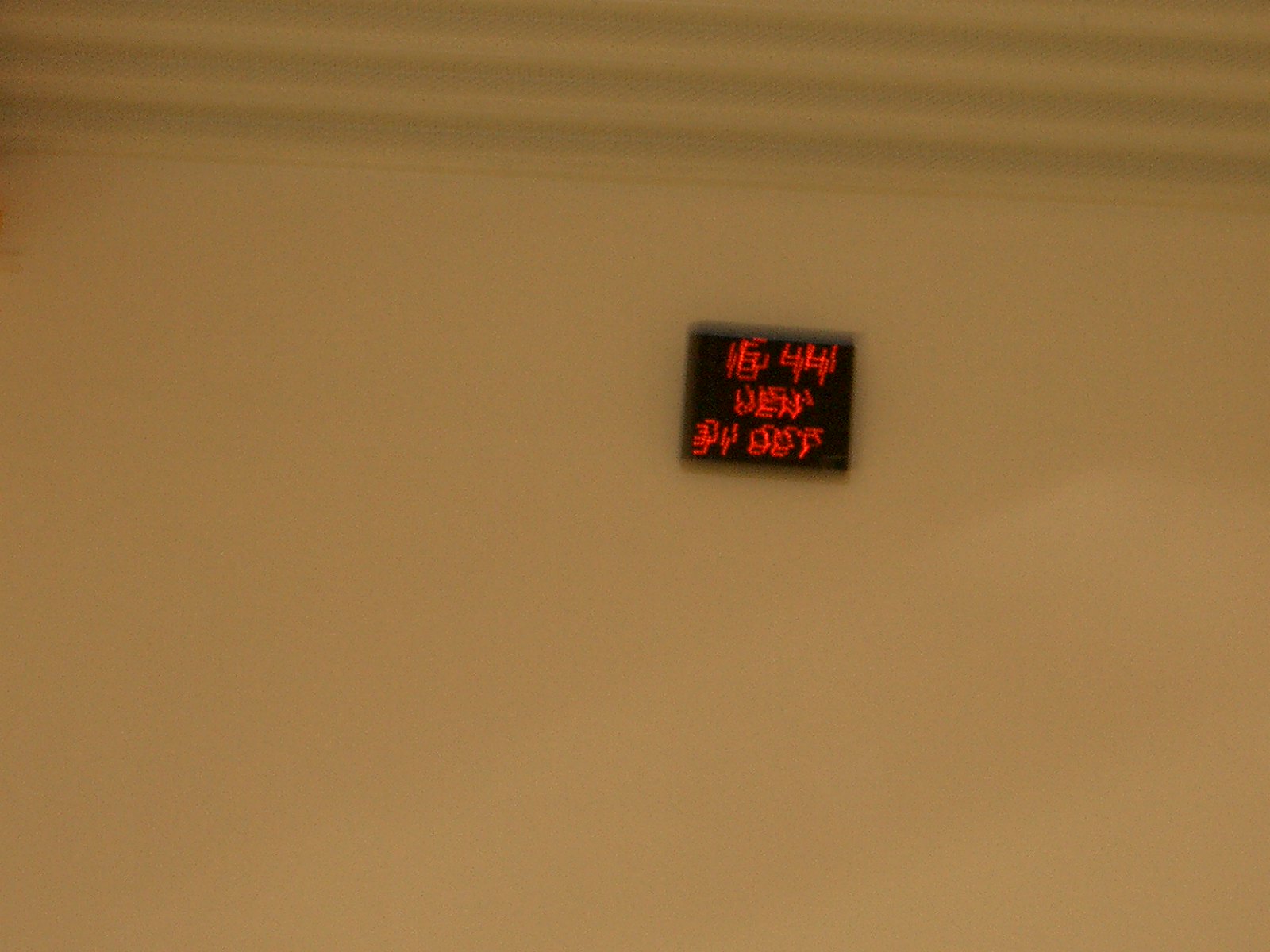A slightly blurry and out-of-focus color photograph of an off-white wall is depicted. The visible portion of the wall showcases a decorative crown molding at the top, characterized by a convoluted surface and divided into three curved, lateral sections. The topmost trim adds an elegant touch to the otherwise plain wall. Affixed to the wall appears to be a small, black sign with red, illuminated text. The text is difficult to discern due to the blur, but it seems to display the numbers "644" followed by some indistinct characters, possibly the abbreviation "OCT," suggesting a date or time. The sign might be a digital clock, though the image’s blurriness makes a precise identification challenging.